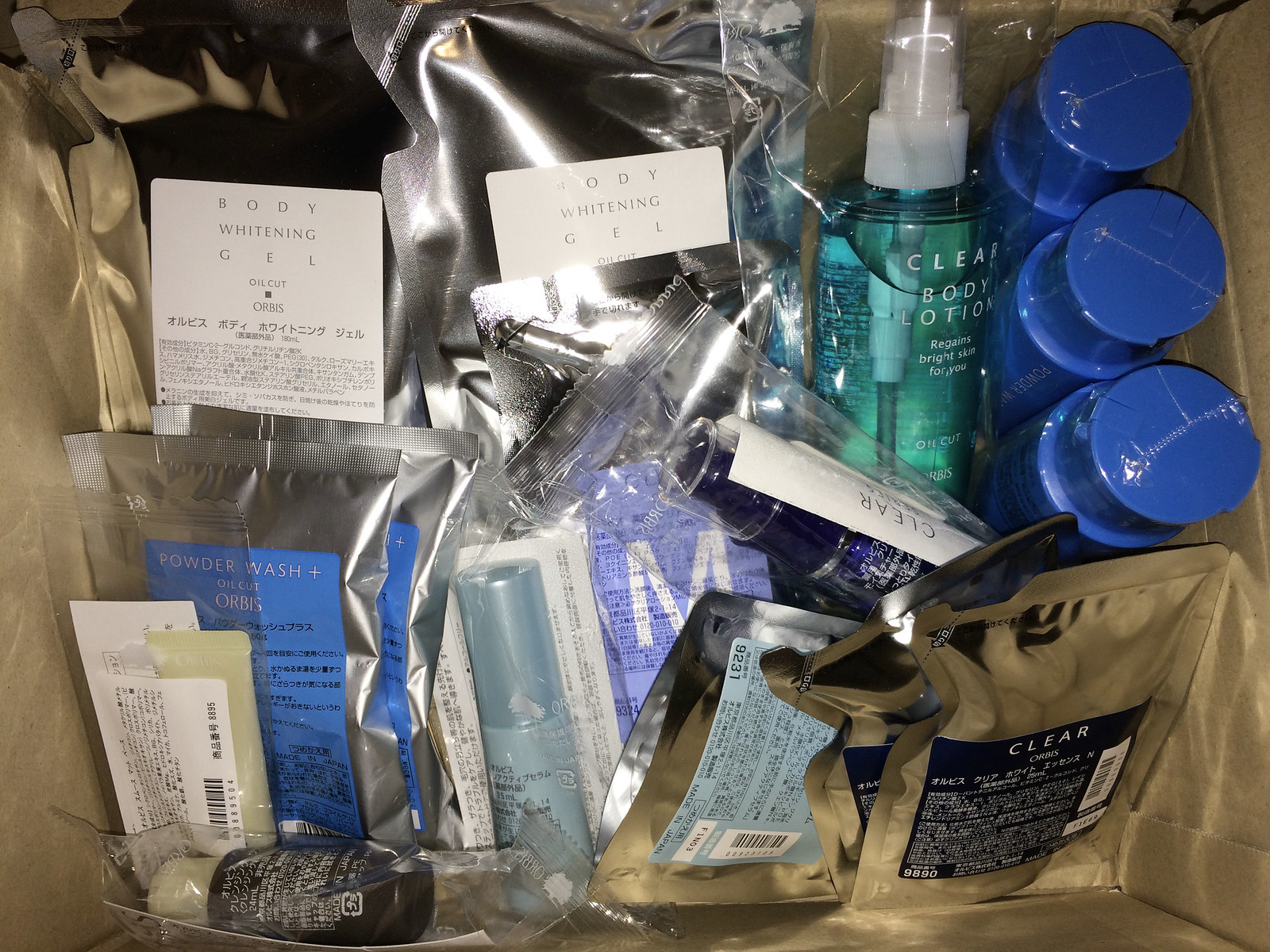The image depicts a specialized kit, meticulously organized for a specific task, though its exact purpose remains ambiguous. The kit features a diverse array of items, each individually packaged. Among the contents, there are three containers resembling either spray cans or containers with screw-top lids. A clear bottle, labeled "Clean Body Lotion," stands out with its pale green liquid and white spray top. Additionally, the kit includes various bottles and bags filled with sprays, lotions, potions, powders, and two items labeled "whitening." Notably, there are hypodermic syringes encased in a sachet. The assortment of specialized components suggests this kit is designed for a precise, albeit unclear, application.